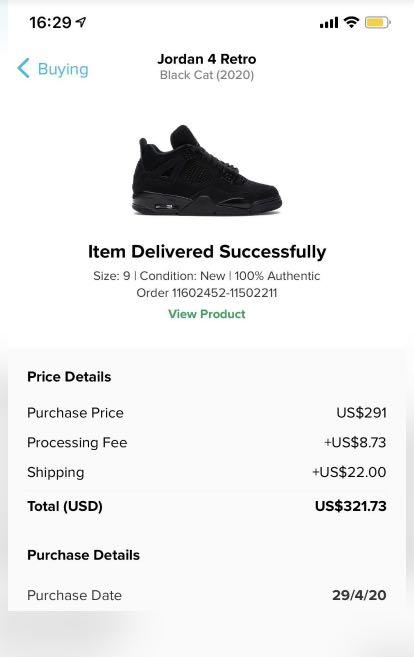This is a vertical image captured on a smartphone device. The backdrop features an ombre effect, transitioning from a darker gray at the bottom to a lighter gray at the top. At the very top of the image, the status bar displays "16:29" on the left, and on the right, there are symbols for full signal strength, Wi-Fi connectivity, and a yellow battery icon. 

On the left side, just below the status bar, there's a blue arrow pointing to text that reads "Buying." Centrally positioned in bold black text is "Jordan Fort Retro," followed by a less bold "Black Cat 2020." Below this, there is an image of the black sneaker, beneath which it is stated, in bold, "Item delivered successfully." Further down, lighter text notes "Size: 9, Condition: New, 100% Authentic," along with an order number.

In green, there is a clickable "View Product" button. Adjacent to this is a gray rectangular box with the bold heading "Price Details." Underneath, in less bold text, it lists "Purchase Price," "Processing Fee," and "Shipping Total." Beside each cost, "USD" is bolded. 

Additionally, "Purchase Details" is in bold, with the purchase date provided as "29/4/20," also bolded. The purchase price is listed as "291 USD," the processing fee as "8.73 USD," and the shipping cost as "22 USD," culminating in a total of "321.73 USD."